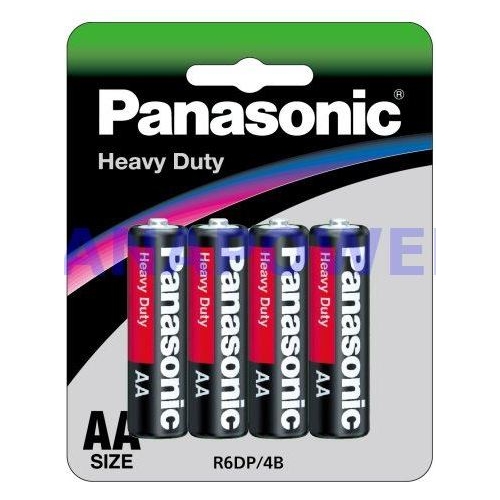The image depicts a package of four Panasonic heavy-duty AA batteries. Each battery is encased in a black exterior and prominently marked with "heavy-duty" written vertically along their sides, as well as "AA" indicated near the bottom. The tops of the batteries feature a silver chrome area that contrasts with the black body.

The packaging itself boasts a distinctive design. The upper section is a solid strip of green, which transitions into black as you move downward. A dynamic swoosh runs across the middle of the packaging, starting pink on the left, shifting through purple, and ending in blue, with hints of green blending in. This colorful swoosh divides the black background of the packaging, leading to a gray section at the bottom. This gray area serves to highlight the black batteries, making them stand out more.

At the very bottom of the package, centered and printed in black capital letters, is the product code "R6 DP / 4-B."